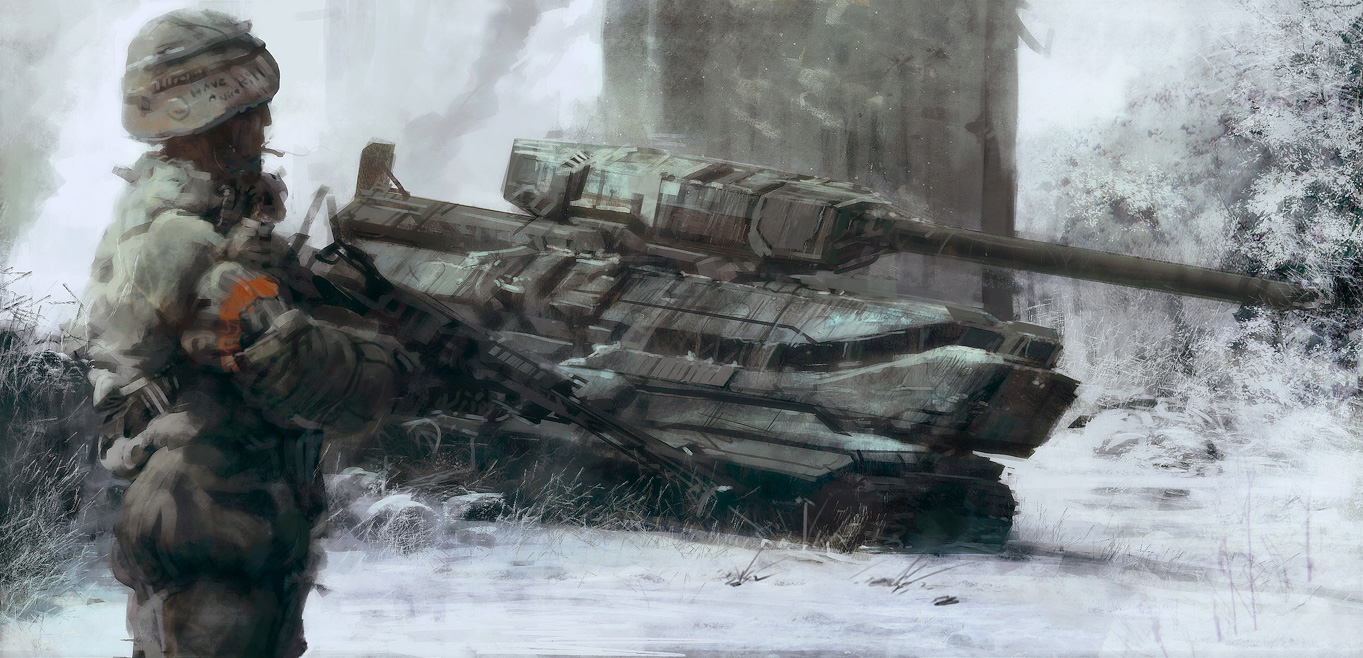The image depicts a detailed war scene rendered in black and white, possibly through a stencil or pencil drawing technique. At the forefront stands a soldier clad in an army uniform and helmet, clutching a large machine gun with a cigarette hanging from his mouth. An orange, possibly red, armband adorns his upper arm, adding a striking contrast to the monochrome palette. The soldier's gaze is directed towards a large, imposing tank in the background, which seems to be either operational or slightly run-down. The tank, box-shaped with intricate line details, appears to be moving or poised to roll over a snowy hill. The entire scene is set against a wintry landscape, where sparse foliage and ground are blanketed in snow, creating an atmosphere of cold desolation. The meticulous depiction of the tank and the soldier's determined posture suggest a moment of intense anticipation or preparation amidst a grim battlefield.